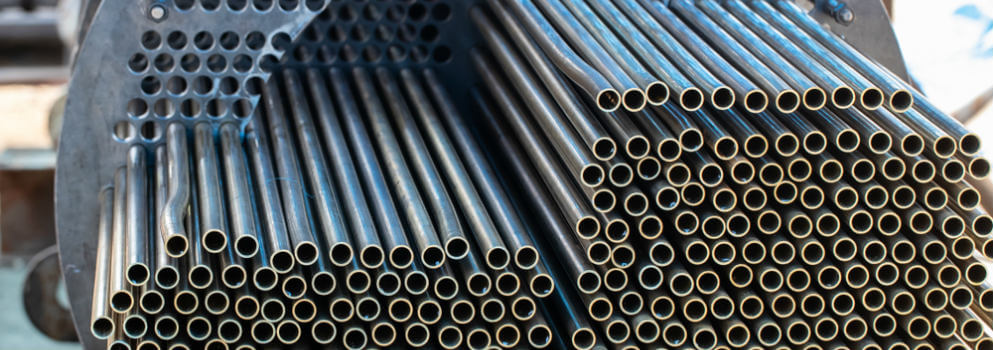This landscape-mode photograph captures a meticulously arranged stack of silver metal pipes, likely steel, organized within an intentional framework. The setup features a circular frame with cutouts, through which the pipes extend. The array includes two distinct but close piles of tubular structures, with the left stack being shorter and the right stack about twice as tall. There are approximately 20 to 25 pipes per row, stacked up to 10 rows high, though not uniformly, suggesting some have slightly shifted. The flat, front ends of the pipes appear as black circles bordered by goldish-yellow rings due to the lighting, while the pipes shrouded deeper in the structure maintain their silver hue. A metallic screen with a notable rip in the top left-hand corner is also part of this holding assembly. The background transitions from dark gray to yellow, then to dark gray again and finally to a light blue at the bottom left. The top right corner of the image is illuminated with bright light, though the source is obscured.